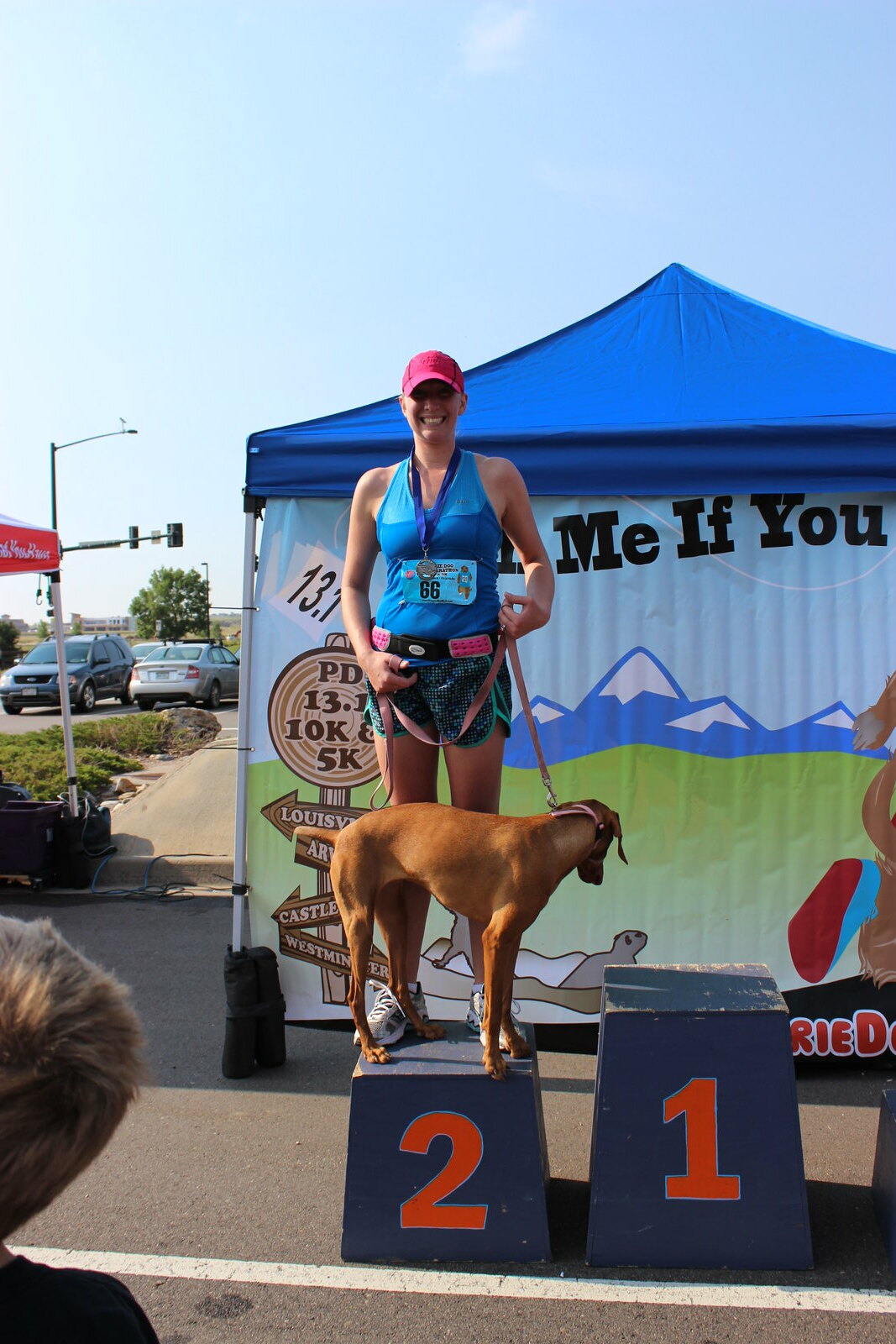In this vibrant outdoor summer scene, a woman stands proudly on a purple pedestal marked with the number "2," indicating her second-place finish in a dog show or race competition. Dressed in a sleeveless blue shirt and black shorts with turquoise trim, she sports a red baseball cap that shades her light-skinned face. Around her neck hangs a black lanyard with a competition number tag attached. By her side is her brown dog with floppy ears, sitting obediently. Immediately to her left is a taller pedestal labeled "1," currently unoccupied. Behind her, a pop-up tent adorned with a mountain scene provides a picturesque backdrop. The far background reveals several parked cars, a lamppost with traffic lights, and a directional post displaying information about PD, 10K, and 5K races. A blonde spectator's head is partially visible in the lower left corner of the image, capturing a moment of calm in the midst of the event's activity.